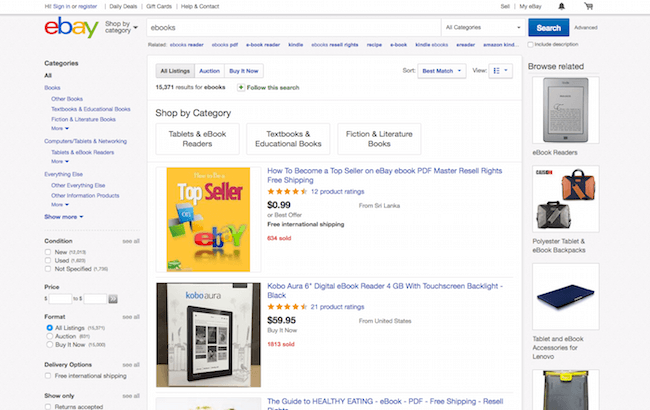This image captures a screenshot of an eBay webpage. The top left corner prominently displays the colorful eBay logo with each letter ("E", "B", "A", and "Y") in a different hue. At the very top of the page, there are hyperlinks allowing users to sign in or register. Adjacent to these options are links for Daily Deals, Gift Cards, and Help & Contact.

Further to the right, options for selling items and accessing the user's eBay account ("My eBay") are visible, accompanied by bell and shopping cart icons. Below this header, there is a search bar where the term "e-books" has been entered.

The page displays two listings for e-books: the first is titled "How to Become a Top Seller," an eBay e-book in PDF format with master resell rights, featuring a five-star rating. The second listing is for a "Kobo Aura 6” Digital E-Book Reader," boasting 4GB of storage, a touchscreen, and a backlight. This item is priced at $59.95 and has received 21 product reviews.

On the left sidebar, there are various filter options, allowing users to refine their search by condition, type of book, pricing, and delivery options. To the right of the listings, there is a section to browse related book items. This organized layout provides users with multiple ways to navigate and optimize their shopping experience on eBay.